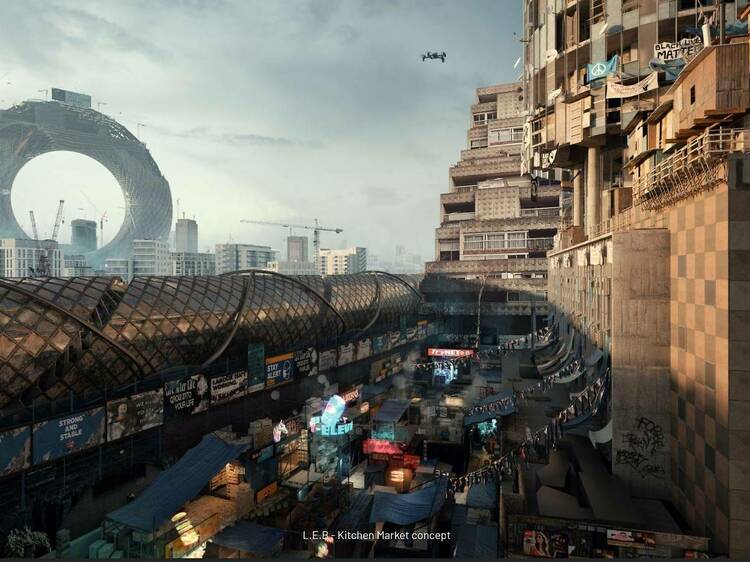The computer-generated image presents a futuristic, somewhat dilapidated cityscape under a gray, cloudy sky, suggesting a scene from a video game. Dominating the background is a prominent donut-shaped building, or circular structure, that hints at advanced architectural designs. Below, on the left side, a large cylindrical tube, potentially a high-speed transportation system, snakes through the city. To the right, tall, weathered apartment buildings with makeshift balcony structures and numerous windows line the scene, interspersed with billboards, including one displaying a "Black Lives Matter" message. Alongside the buildings, strings with hanging items and wires bind a visible pipeline, contributing to the makeshift, shantytown atmosphere. At street level, stalls and a possible refugee camp signify a bustling yet struggling community. The lower part of the image features white text that reads, "LEB Kitchen Market Concept," indicative of an urban market area within this complex, multi-layered environment.